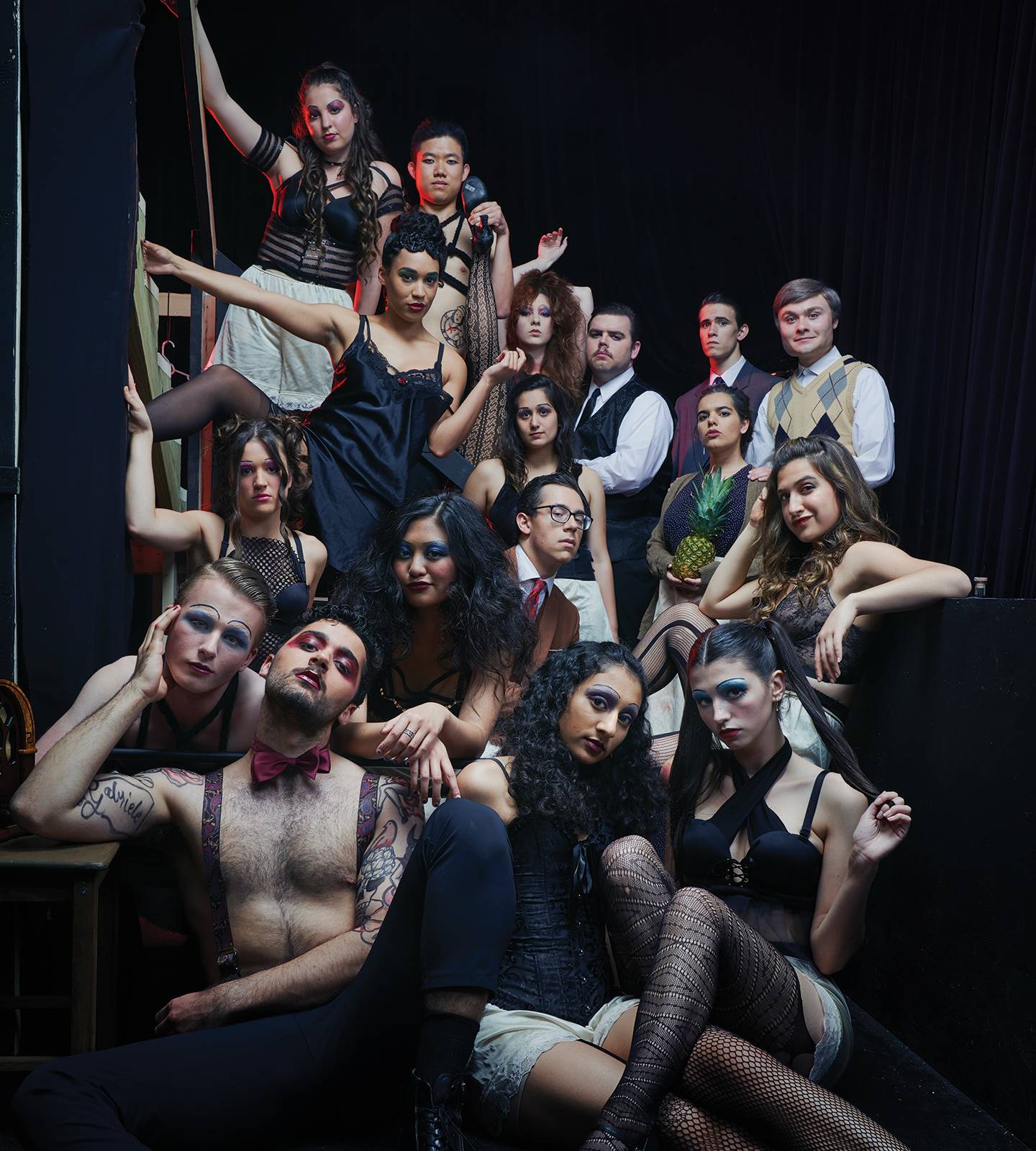In this photograph with a black background, we're likely looking at a theatrical cast posing for a picture. The scene is quite striking, featuring around 20 people, both men and women, intricately grouped together. The front row is notable for its audacious style, with shirtless men wearing just suspenders and bow ties, their faces adorned with heavy, dramatic eye makeup in vivid colors like bright blue and red, extending past their brows and onto their cheeks. Around them, women in skimpy clothing and heavy eyeliner lean against one another and the men, creating a visually cohesive yet eclectic group.

Behind this front row, the diversity in attire becomes even more apparent. Some men are more traditionally dressed, sporting suit jackets, ties, and sweater vests with their hair slicked back. On the top left, several men and women don nightgowns and pajamas, contrasting sharply with the more scantily clad individuals below. In the midst of this unusual assembly, one woman stands out, holding a pineapple, adding an unexpected quirk to the composition. The whole group, with their varied and eccentric outfits, all direct their gaze towards the camera, striking a collective pose that emphasizes the theatrical and flamboyant nature of the scene.